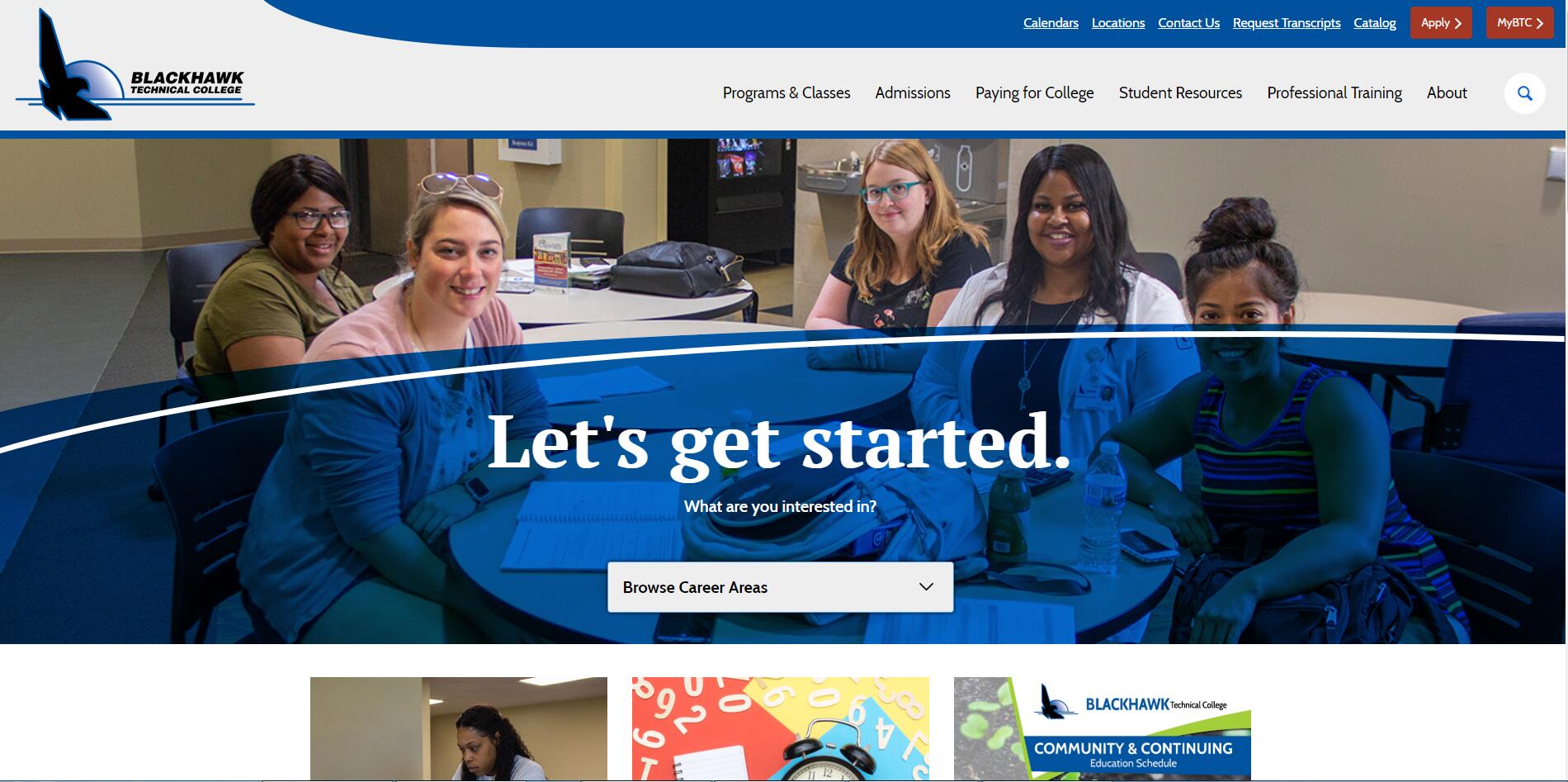The website features the homepage of Black Hawk Technical College, prominently branded with the institution's logo in the upper left corner. The logo consists of a black silhouette of a hawk in flight, set against a stylized backdrop that fades from blue to white, forming half a circle with two lines beneath it. The text "Black Hawk Technical College" is displayed in black on a white background.

At the very top of the website, there's a horizontal blue bar containing navigational links: "Calendars," "Locations," "Contact Us," "Request Transcripts," and "Catalog," all in white font with underlines, indicating they are clickable. To the right of these links are two prominent red buttons with white text – one labeled "Apply" and the other "myBTC."

Beneath this, the main navigation menu appears, offering links to "Programs and Classes," "Admissions," "Paying for College," "Student Resources," "Professional Training," and "About." A search icon with a magnifying glass is also present for easy access to the site's search functionality.

The central portion of the page is dominated by a background photograph over which the text "Let's Get Started" is displayed in white. Below this slogan, there is a prompt reading "What are you interested in?" also in white. A dropdown menu labeled "Browse Career Areas" allows users to explore various fields of study, helping them to navigate through the college's offerings.